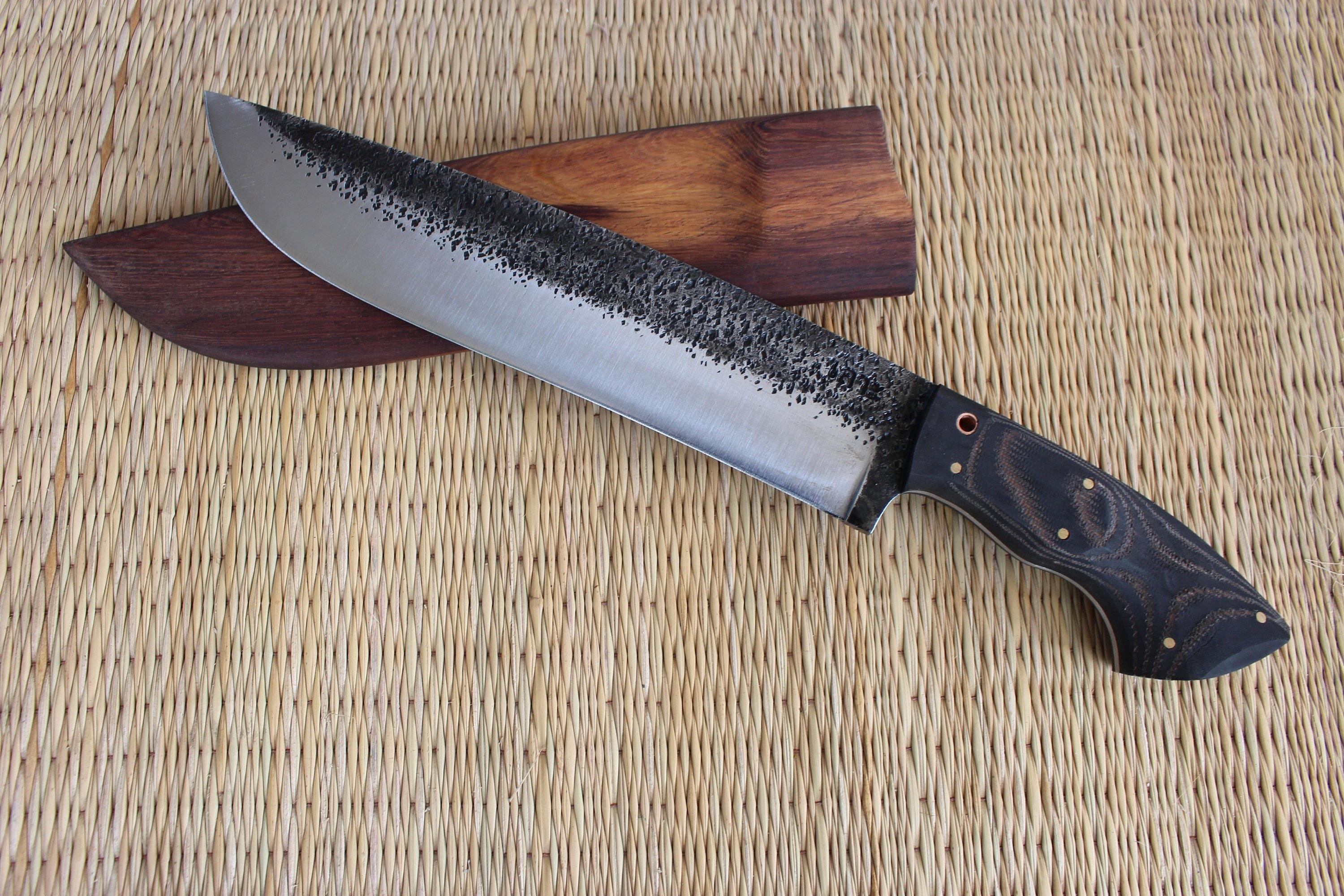This detailed image captures a knife and its wooden sheath placed atop a woven beige mat resembling a wicker or bamboo style. The knife is positioned at a 35-degree angle to the bottom of the photograph. The knife handle is black with light brown streaks and dotted with small yellow or gold marks. The blade, a wide design tapering to a point, is variegated with the bottom half in silver and the top half in speckled, rough-textured black, giving a rusted or corroded appearance. The blade lies across an intricately crafted wooden sheath, which exhibits a fine grain and variegated coloring, transitioning from dark brown at the bottom to lighter brown towards the top and middle. The sheath mirrors the shape of the knife blade and suggests an air of craftsmanship and expense. The background mat provides a contrasting textured surface, highlighting the knife and sheath's detailed and refined features.